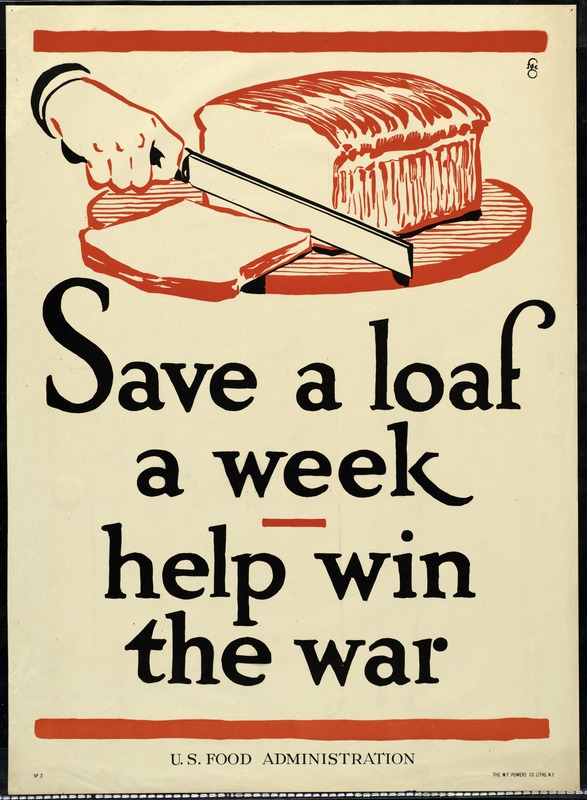The image is an old advertisement with a rectangular, vertical layout and black borders. The background paper has a yellowed tone suggesting age. At the top and bottom of the flyer, there are long red horizontal bars. Beneath the top bar, there's a red sketch of a loaf of bread being sliced by a hand holding a knife. The sketch includes a wooden turntable beneath the bread. Below this image, the text reads in bold black font over four lines: "Save a loaf a week. Help win the war." At the very bottom of the flyer, another red horizontal bar frames the smaller black text that says, "U.S. Food Administration," with some fine print in the bottom right corner. The major colors in this image include orange, brown, black, and shades of yellowed paper.